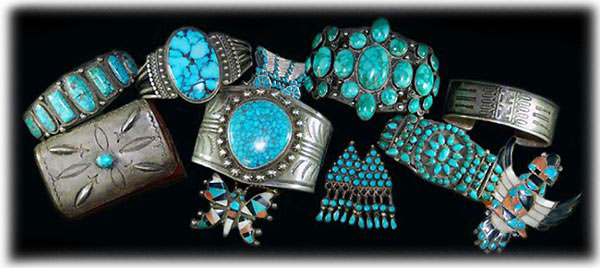This indoor close-up photograph features a collection of intricately designed jewelry displayed against a completely black, slightly hazy background. The assortment includes six or seven items predominantly showcasing various shades of blue stones, akin to turquoise or Tiffany blue. On the left, a bracelet adorns a Tiffany blue stone, while on the right, a ring features a central, marbleized blue material. Another bracelet on the right is embedded with multiple blue stones. The bottom right displays a piece, potentially a pendant, depicting an Azteca bird with multicolored stones. Also prominent are earrings with a pyramid pattern, and a majestic gauntlet with a prominent marble Tiffany blue rock. Additionally, a small butterfly-shaped brooch and a piece resembling a bug adorned with multicolored stones are visible in the center and foreground, respectively. The intricate designs and silver craftsmanship of these pieces evoke a sense of elegance and detailed artistry.